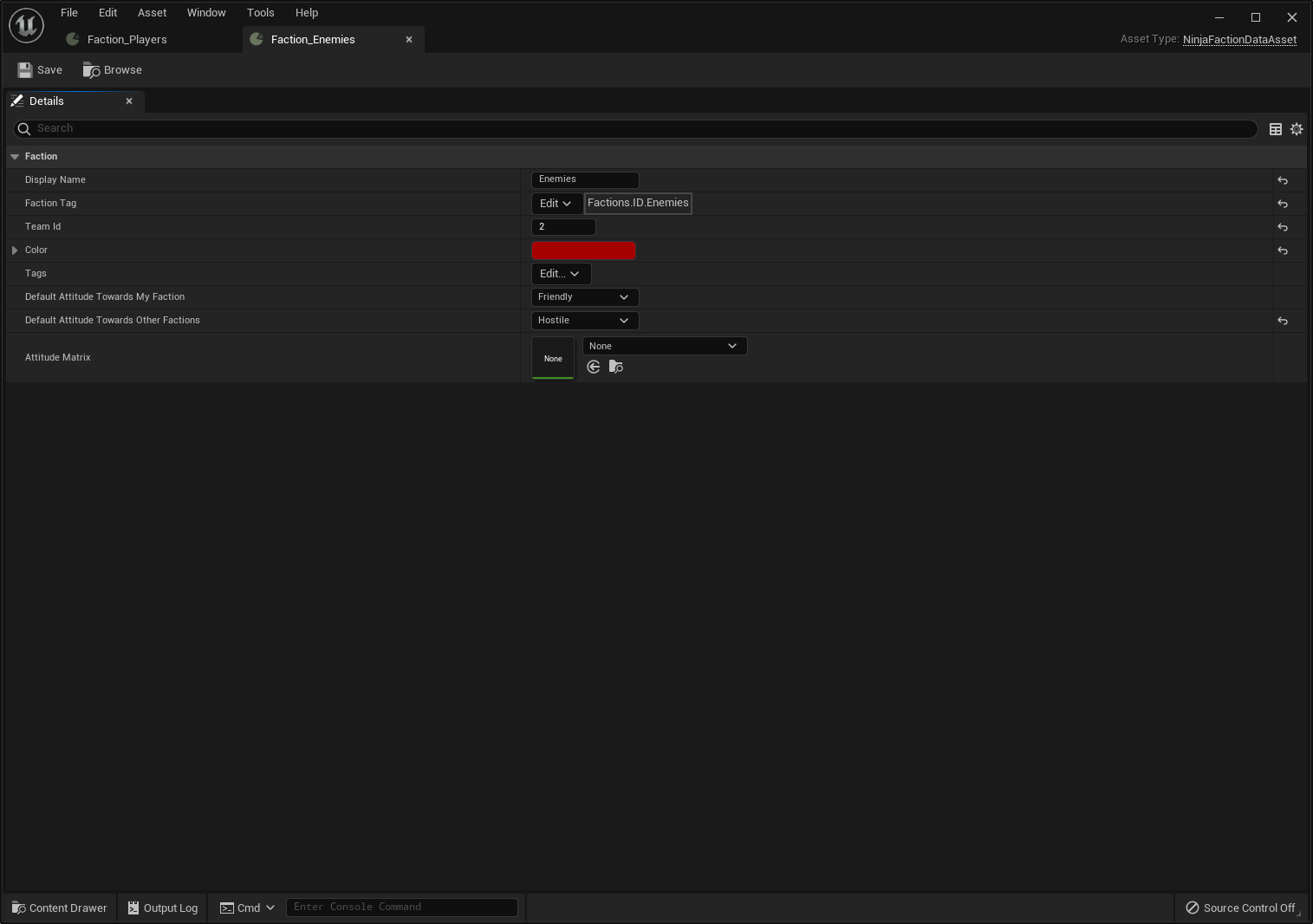The image displays a software application with a predominantly black background. Despite the small font, various interface elements are clearly distinguishable. In the upper left corner, there's a prominent black circle with a white ring encasing an icon of two vertical lines. The top menu bar includes the options: File, Edit, Asset, Window, Tools, and Help, with Minimize, Maximize, and Close buttons on the upper right.

Directly below the menu, there are two open tabs labeled "Faction Players" and "Faction Enemies," with the latter being highlighted. Below these tabs, the interface displays buttons labeled "Save" and "Browse," followed by a section titled "Details" accompanied by a small 'X' icon. 

Further down, there's a search function and a dropdown menu. Adjacent to the dropdown are fields labeled: Faction, Display Name, Faction Tag, Team ID, Color, Tags, Default, and another unreadable field. There is also a section titled "Attitude Matrix."

At the very bottom of the application window, a banner spans the width of the interface, containing text that is unfortunately too small to decipher. The overall design suggests the application is meant for managing factions within a game or simulation, possibly used for development purposes.